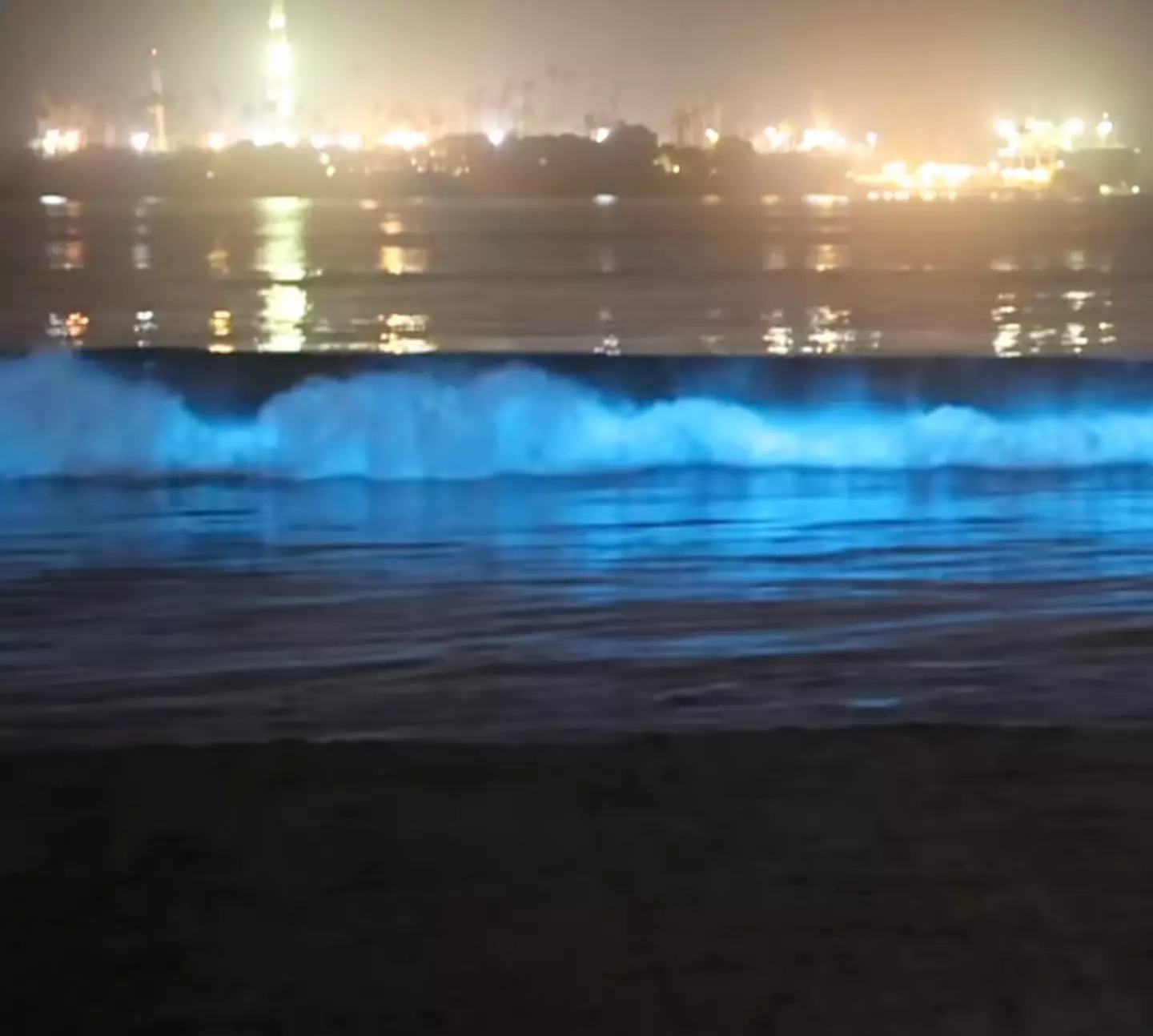This nighttime photograph captures the mesmerizing phenomenon of ocean bioluminescence. The grainy texture suggests it was likely taken with a low-resolution camera, possibly a webcam. The focal point of the image is the ocean, with waves rolling in and crashing onto an indistinguishable beach, creating luminous blue highlights that reveal the bioluminescent effect. The scene is set against a backdrop of a vibrant, illuminated pier. The lighting from the buildings on the pier is so intense it creates the illusion of a fiery glow, though this is merely the result of light glare captured by the camera. One building, taller than the rest, stands out near the left edge, its lights rising higher into the sky. Palm trees are faintly visible, adding a tropical touch to the setting, which appears to be a bustling coastal area, possibly a bay or island. The absence of boats creates a serene, almost still water surface, except for the dynamic crashing waves. The beach itself fades into darkness, making it difficult to distinguish specific details, emphasizing the dramatic interplay between light and shadow in this captivating scene.